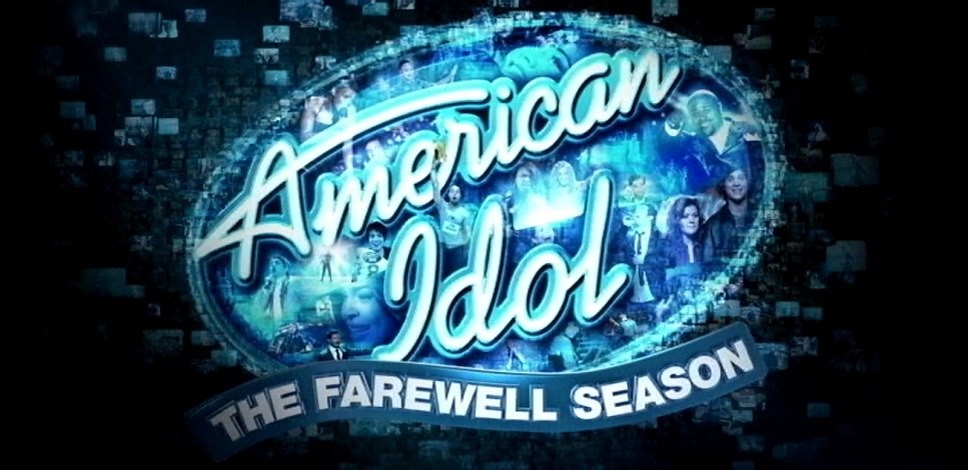This digitally produced image, likely a logo for television or a website, prominently features the "American Idol: The Farewell Season" text. The predominant colors include black, light blue, dark blue, white, and gray. The central focus of the image is a logo, placed directly in the middle, featuring the "American Idol" title in a white font with a blue border. Below this, a blue banner with white text reads "the farewell season." The logo is composed of various smaller images, possibly related to moments from the show, with the background depicting a black scene with what appear to be smaller screens or picture fragments flying outward. Among these images within the logo, Kelly Clarkson is notably recognizable. The design gives an impression of the logo disintegrating, with pictures seemingly drifting into the background, echoing the theme of the final season of "American Idol."